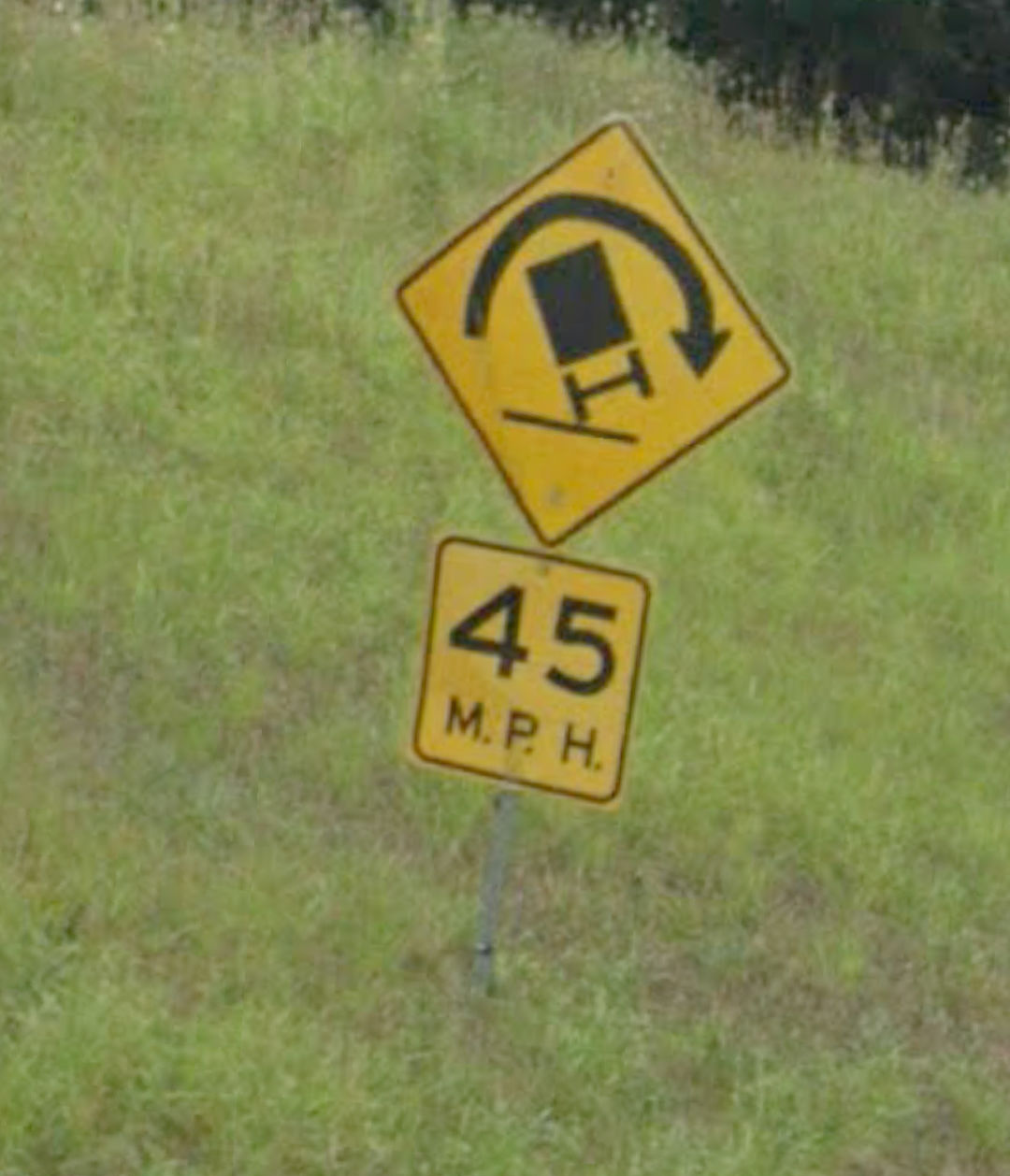The image depicts two traffic signs mounted on a single post in a grassy field with tall, unkempt green weeds. The top sign is triangular, featuring a yellow background with a black border. It illustrates a truck on a steep grade, with its right wheels off the ground, and an arrow curving from left to right, indicating a rollover hazard. The truck icon shows a separate cab and cargo box with a barbell-like hub for the axle, emphasizing the risk of tipping. The bottom sign is rectangular and indicates a speed limit of 45 miles per hour in black print. The field surrounding the signs is lush but appears neglected, adding a sense of isolation to the area.